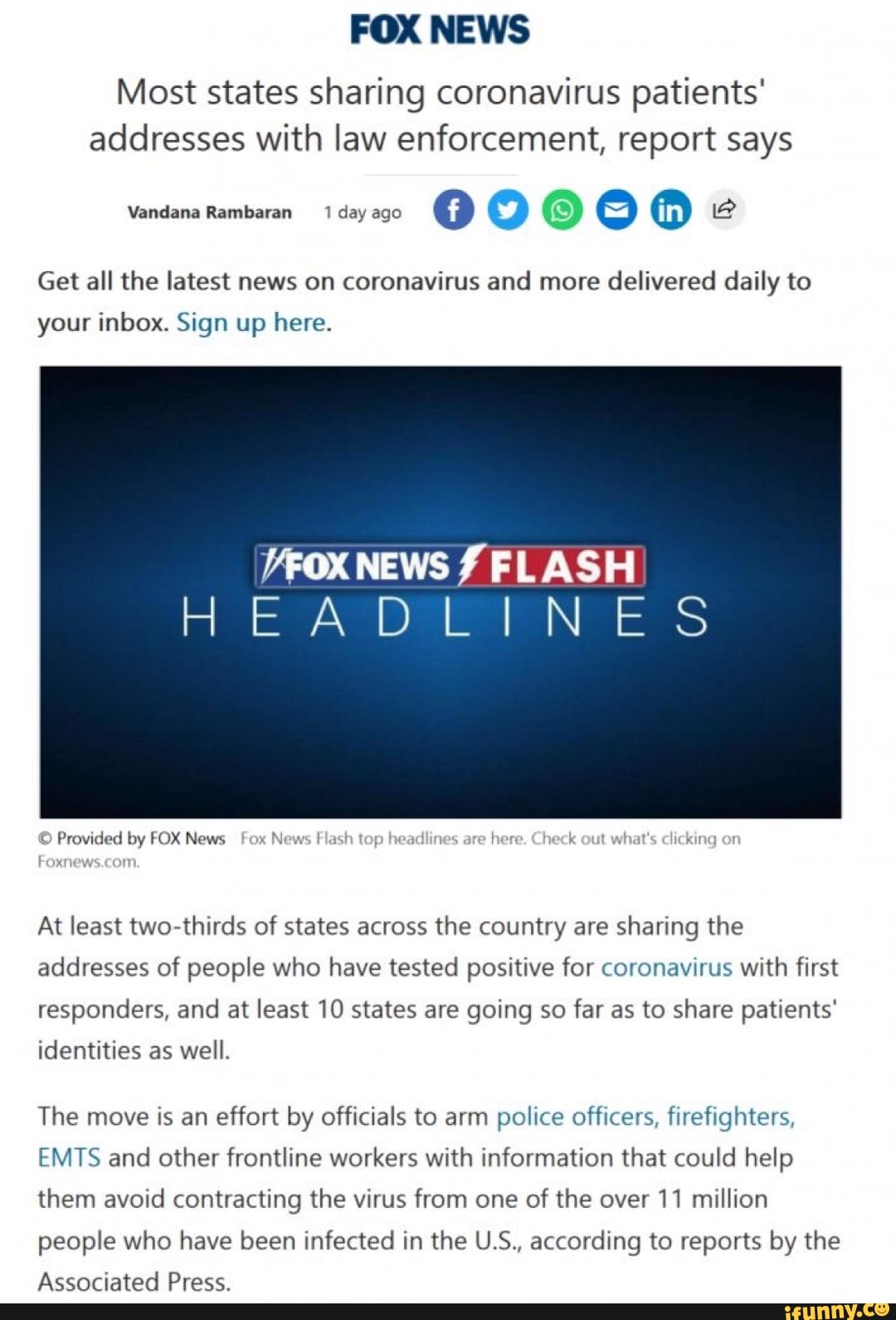A recent report reveals that the majority of U.S. states are sharing the addresses of individuals who have tested positive for COVID-19 with law enforcement agencies, according to Fox News. This initiative aims to protect first responders—including police officers, firefighters, and emergency medical technicians (EMTs)—by providing them with critical information to help avoid contracting the virus as they carry out their duties. Notably, at least ten states have extended this measure to include sharing patients' identities. This development comes amidst efforts to curb the spread of the virus, which has already infected over 11 million people in the United States. For more updates on the coronavirus and other news, visit foxnews.com. Information sourced from the Associated Press and Ifunny.co.